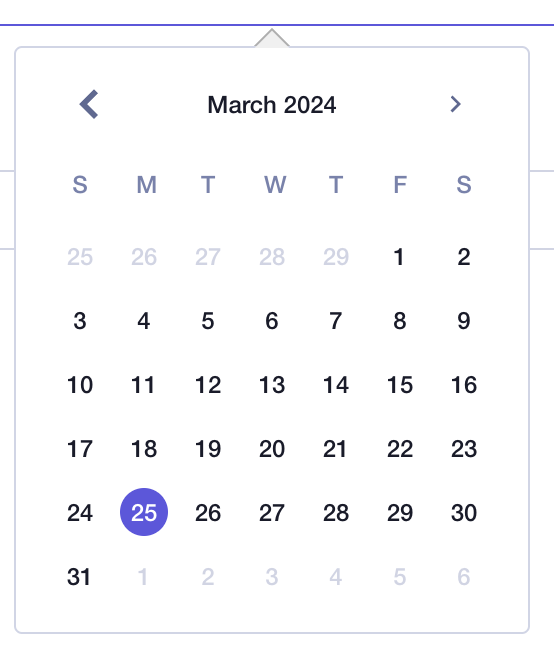This screenshot captures the interface of a mobile device, showcasing a calendar application with a distinct white and purple color scheme. The image features a vertically elongated layout, typical of a cell phone's dimensions. 

At the top of the screen, a purple banner with white text prominently displays the date "Tuesday, April 18th, 2023" in a somewhat repetitive format: "2023-2-TUE-Tuesday-April-Apr-Apr-2-Apr-18." Directly below this banner, the main calendar interface is visible with a white background and black text.

Centered within the calendar display, the current month "April 2023" is indicated, flanked by left and right arrows allowing for navigation to previous and subsequent months. Below the month header, the days of the week are abbreviated as Su, Mo, Tu, We, Th, Fr, and Sa, representing Sunday through Saturday respectively.

The calendar layout reveals that April 2023 begins on a Saturday, with the number "1" positioned at the far right of the row. The date "18th April 2023" is distinguishable by a purple circle, indicating it as the selected or current date.